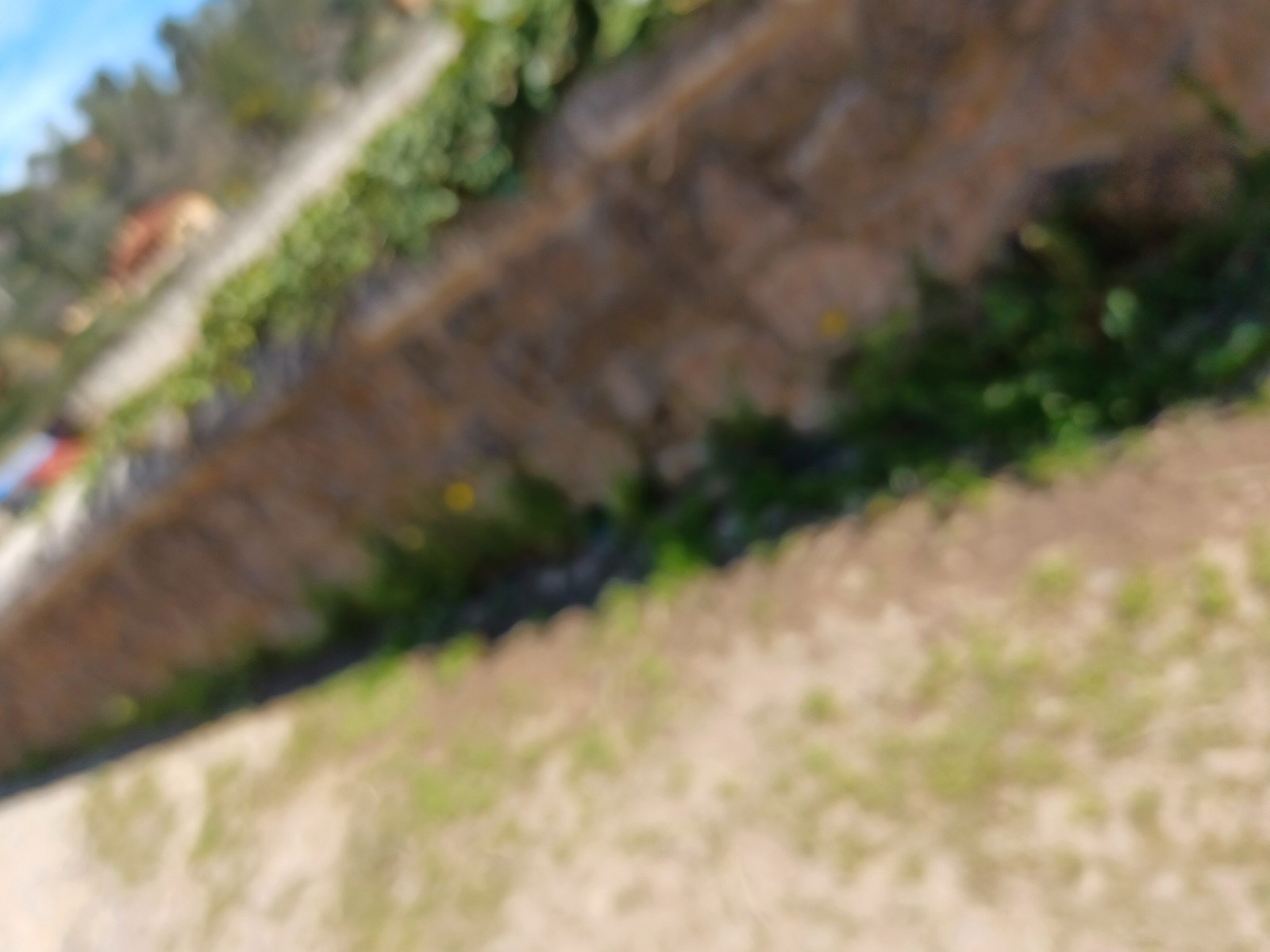The image presents a very blurry outdoor scene taken at a 45-degree angle, looking down. Dominating the foreground is a stretch of discolored cement with elements of tan, brown, gray, black, and orange, possibly a curb or gutter, with weeds and moss growing along its edge. Above this, extending diagonally, is what appears to be a retaining wall or curb constructed from large pieces of stone, partially obscured by greenery, including ivy and weeds, some bearing yellow dandelion-like flowers. The scene beyond is difficult to discern due to the blurriness, but it appears to show a tan area that might be a sidewalk or road and potentially a blurry vehicle or object, perhaps a car or even a yellow building. In the background, there's a vague tree line under a light blue sky dotted with white clouds.